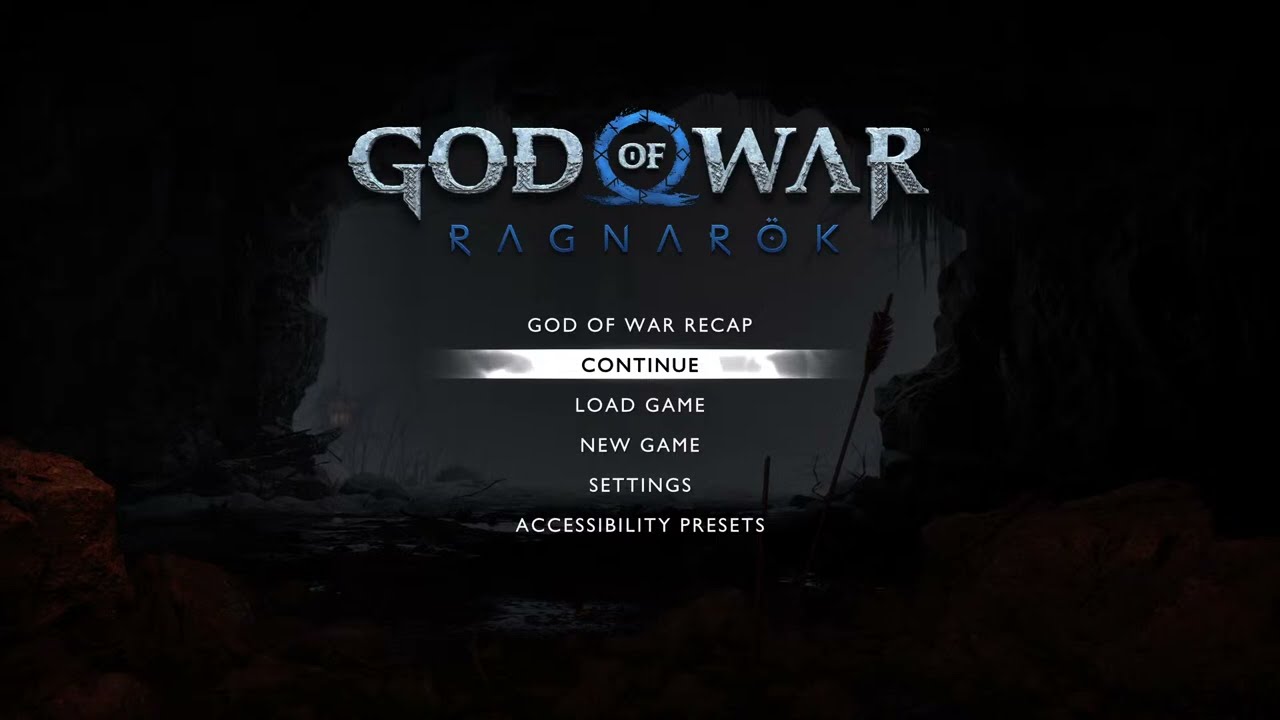This image depicts the main menu of the video game "God of War Ragnarok." The predominant background is black, with a cave-like aesthetic featuring dim lighting, sporadic grass sprouts, a red rock on the far left, and an overall dark ambiance. At the top of the screen, the game's title "God of War" is prominently displayed in bold, metallic gray lettering. The word "OF" is encapsulated within a circular, blue emblem, standing out between "God" and "War." Below the main title, "RAGNAROK" is written in a distinctive blue font.

The menu options listed beneath the title are as follows, all in white text:
- God of War Recap
- Continue (which is highlighted, indicating the current selection)
- Load Game
- New Game
- Settings
- Accessibility Presets

The detailed depiction of the main menu encapsulates the start of the game, setting a gripping tone for the player.